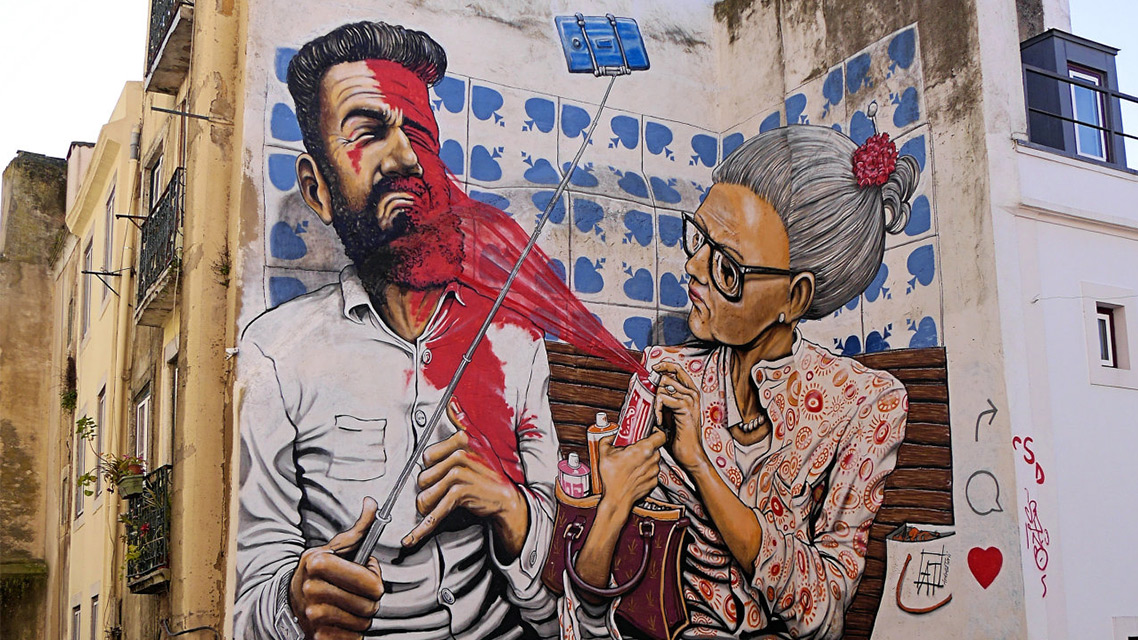The image showcases a multi-story mural on the inside corner wall of an older building in Lisbon, Portugal, known as the "Old Lady of Lisbon." This piece of urban art depicts an older woman with gray hair styled in a bun adorned with a red flower, thick prescription glasses, and wearing a shirt with a circular geometric design and pearls around her neck. She sits on a park bench with a man who has combed-back black hair, a large beard, and is dressed in a white button-down shirt. The man is holding a selfie stick with a phone, capturing a moment as the woman sprays red paint or blood from a can directly onto his face, covering half of it and staining his shirt. The woman has additional spray cans in her tote bag, and the scene is set against a backdrop designed to resemble tiles with blue hearts at each corner. The artwork vividly captures the striking and somewhat humorous interaction between the two characters, making it a standout piece of the local urban art landscape.